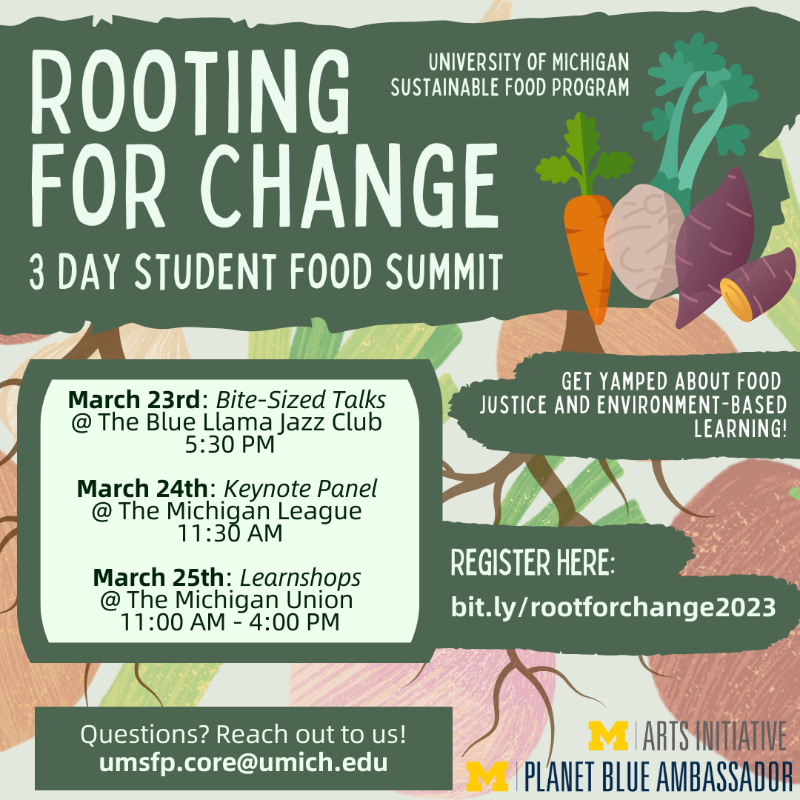The poster promotes the "Rooting for Change: Three Days Food Summit" organized by the University of Michigan Sustainable Food Program. The top features a green background with the headline in white text. Below this, there's a variety of illustrated vegetables, including carrots, turnips, and sweet potatoes. The main slogan reads, "Get Yamped About Food Justice and Environment-Based Learning." 

Details of the summit include:
- **March 23rd:** Bite-Size Talks at the Blue Llama Jazz Club, 5:30 p.m.
- **March 24th:** Keynote Panel at the Michigan League, 11:30 a.m.
- **March 25th:** Learn Shops at the Michigan Union, 11 a.m. to 4 p.m.

For further inquiries, contact umsfp.cor@umich.edu. Registration can be completed at bit.ly/rootforchange2023. The poster also features the University of Michigan logo with a yellow "M," and notes involvement from the Arts Initiative and Planet Blue Ambassador.